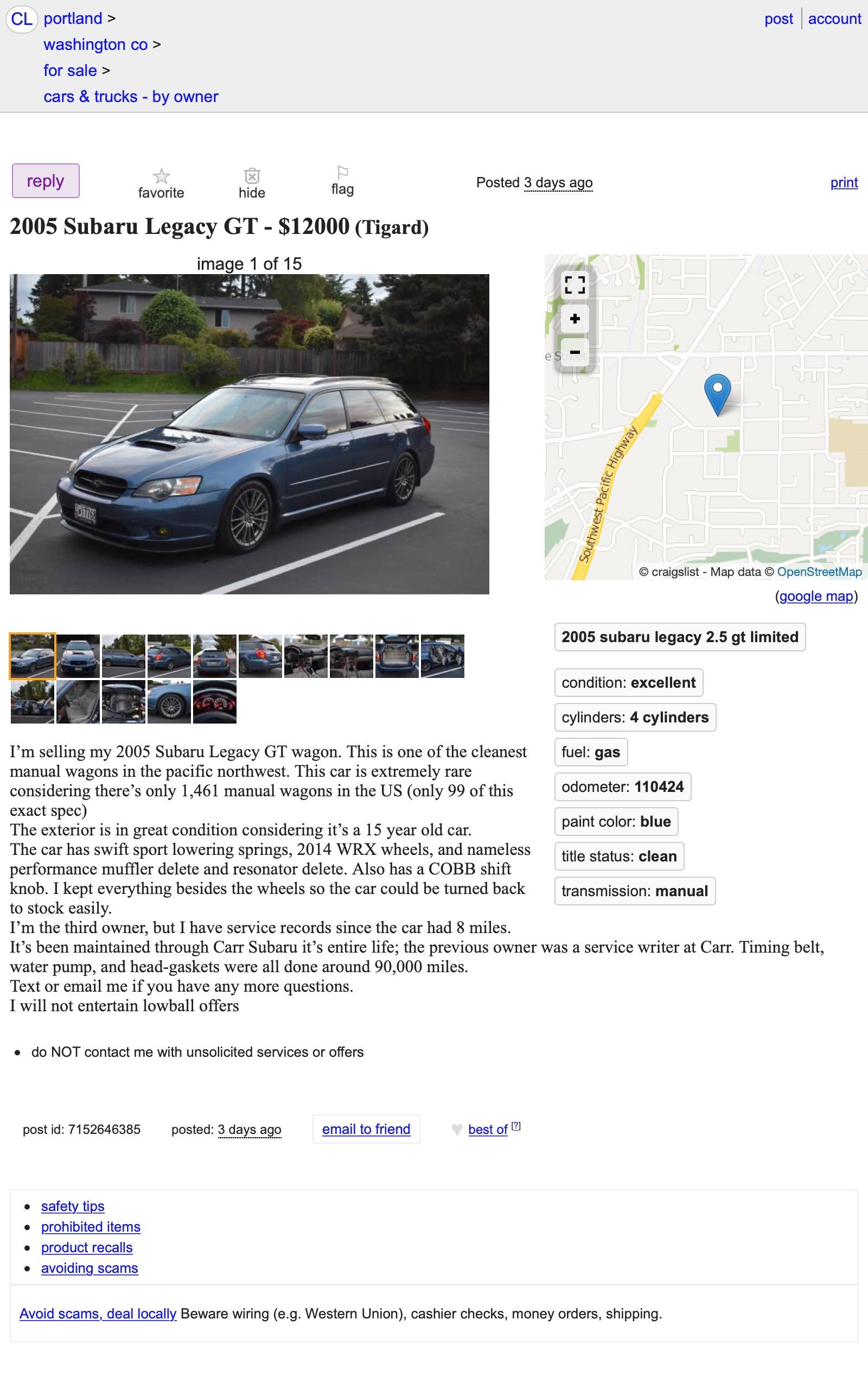"On this image, the top section features text in blue. On the top left, it reads 'Portland, Washington call for sale cars and trucks by owner.' On the top right, there are two blue text links labeled 'post' and 'account.' The main page includes tabs at the top such as 'reply,' 'favorites,' 'hide,' 'flag,' with 'reply' highlighted in purple. 

Beneath these tabs is a photo of a car, a 2005 Subaru Legacy GT, priced at $12,000 and located in Tigard. The image is labeled '1 of 15,' indicating there are 15 images available. The displayed car is slightly navy blue, facing toward the left side, and prominently centered in the image. 

Below the image is a detailed description: 'I am selling my 2005 Subaru Legacy GT wagon. This is one of the cleanest manual wagons in the Pacific Northwest. This car is extremely rare, considering there are only 1,461 manual wagons in the US, with only 99 of these existing in this condition. The exterior is in great condition for a 15-year-old car. It has Swift Sport lowering springs, 2014 WRX wheels, and a nameless performance muffler delete and resonator delete. It also has a COBB shift knob. I kept everything except the wheels, so the car could be easily tuned back to stock. I am the third owner but have service records since the car had 8 miles. It has been maintained by Subaru its entire life. The previous owner was a service writer, and the timing belt, water pump, and head gaskets were all done around 90,000 miles. Text or email me if you have any more questions. I will not entertain lowball offers. Do not contact me with unsolicited services or offers.' The post was made 3 days ago, with options to email the post to a friend and add it to a list of best offers.

At the bottom of the page, several safety tips are provided, including advice on dealing locally, being cautious with wiring and cashiers checks, and avoiding scams. 

On the right side of the page, there is a map indicating the car's current location with a blue pin. The specifications listed include: 
- Year: 2005
- Model: Legacy 2.5 GT Limited
- Condition: Excellent
- Engine: 4 cylinders
- Fuel: Gas
- Odometer: 110,424 miles
- Paint color: Blue
- Title status: Clean
- Transmission: Manual"